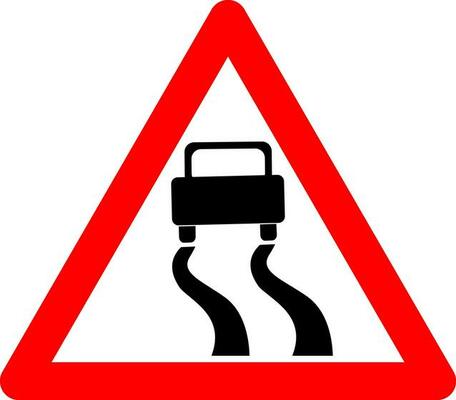This is an image of a triangular road warning sign, depicted in a color illustration with a white background. The sign features a thick red outline on the outermost triangle, which has rounded edges, and a white inner triangle with sharp edges. The central illustration is a black silhouette of a car, positioned horizontally. The car is represented as a black rectangle with an arced line indicating the roof, along with two small curved rectangles at the bottom symbolizing tires. Behind the car, there are black, parallel S-shaped lines suggesting skid marks, indicative of a slippery or slick road warning. The detailed style and elements combine to effectively communicate the hazard through a well-recognized road sign format.